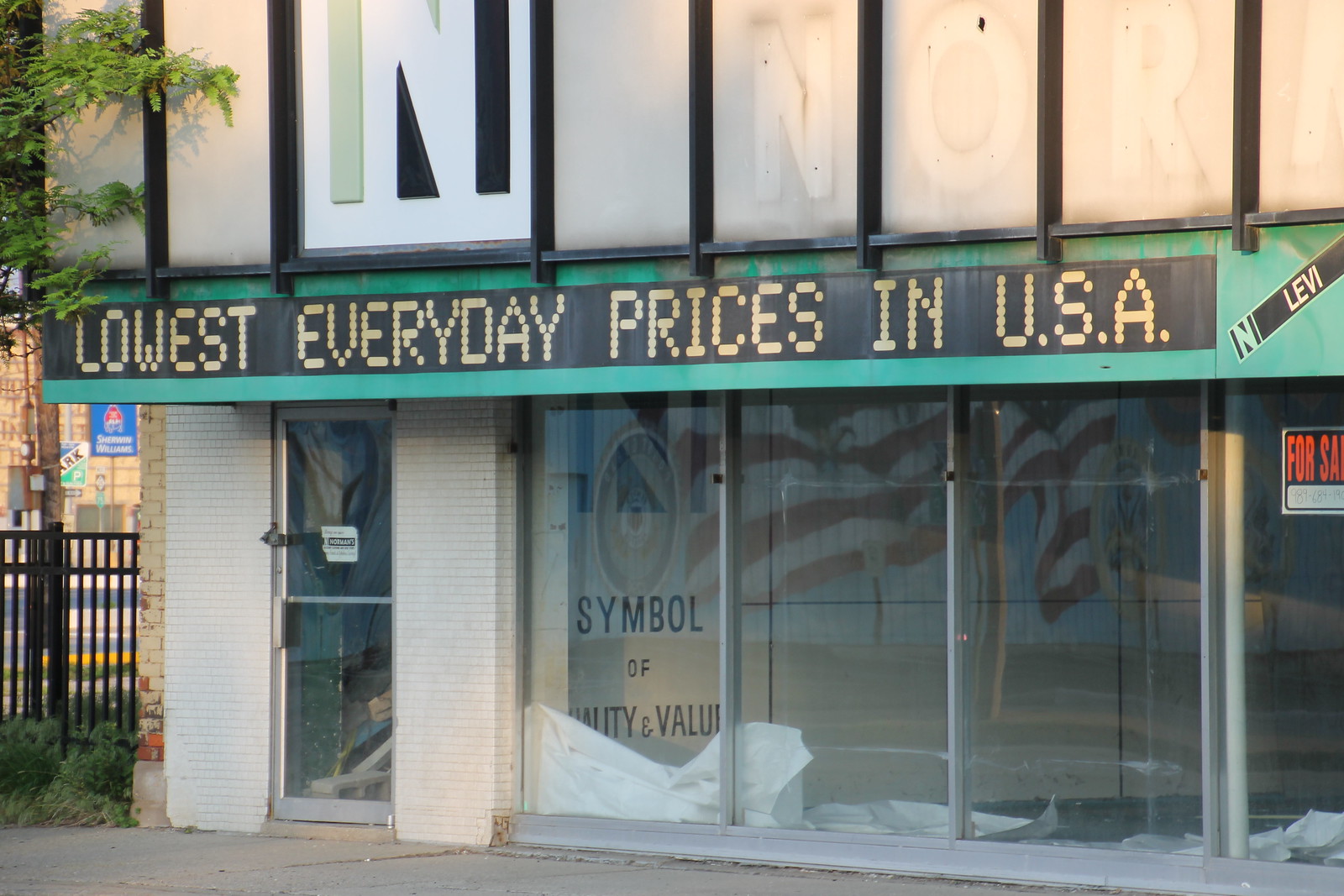This image showcases an empty storefront taken outdoors, featuring a two-level building with prominent glass elements. The ground level is dominated by large plexiglass windows allowing a clear view inside, revealing that the interior is completely cleared out. The entrance is marked by a glass-metal door surrounded by light whitish brick walls. Above the door and windows, a green marquee with black sections and yellow text reads "Lowest Everyday Prices in USA" and includes a partial inscription "N Levi."

To the left of the building, a black wrought iron fence is visible, and a green tree can be seen. The storefront's facade includes vertical black boards against an off-white background, with some sections showing faded outlines of letters where signage once existed, including visible remnants of the letters "N," "O," and "R." Additionally, there is a reflection of an American flag in the windows. On the far right window, an orange block text "For Sale" sign is posted, which also includes a faintly printed phone number. Inside, on the wall, there is painted text that says "Symbol of Quality and Value."